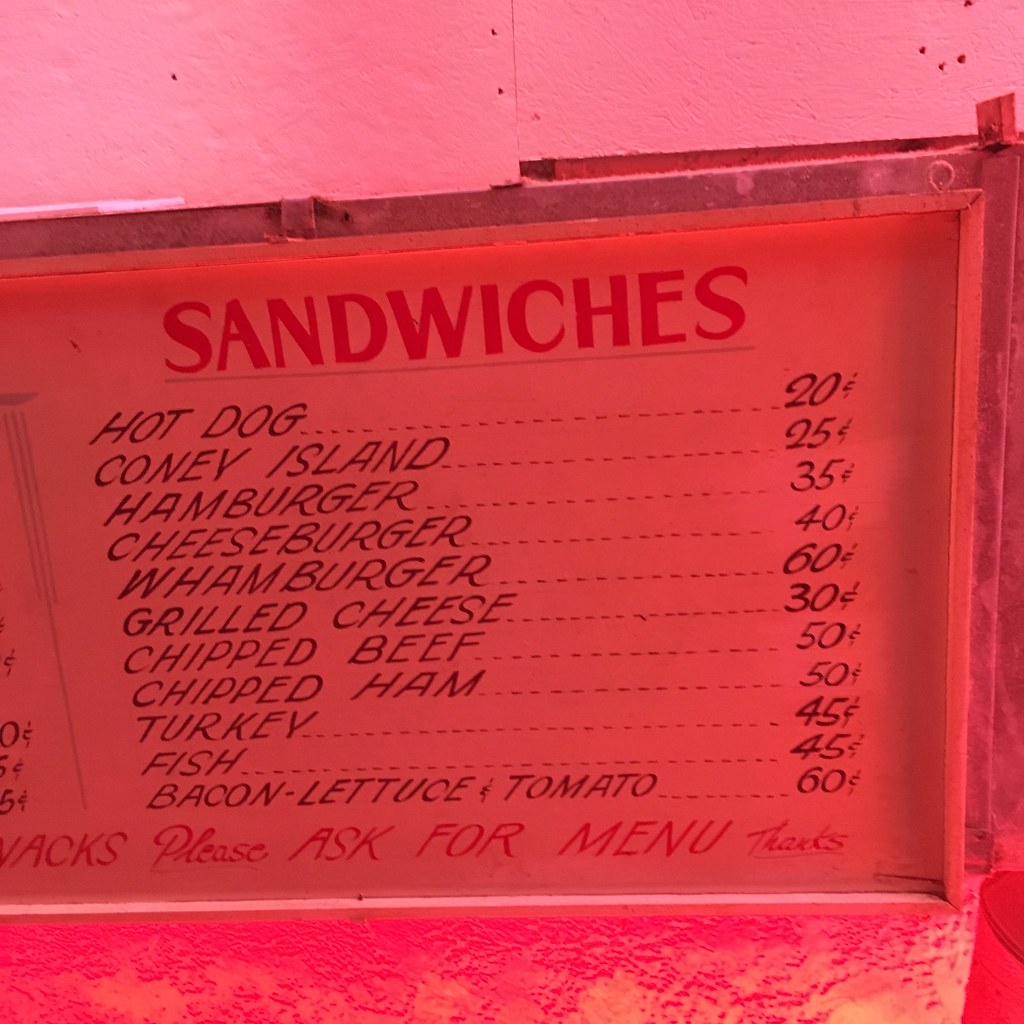This image captures a close-up view of a vintage restaurant menu board, enveloped in a distinct red hue, likely due to a red light illuminating the scene. The menu board itself features a chrome frame and a white background, which accentuates the bold red header reading "SANDWICHES." Below this header, a list of menu items is meticulously detailed in black text, with each item's name followed by a series of dots that lead to its respective price on the right edge. The listed items, starting from the top, include:

- Hot Dog - 20 cents
- Coney Island - 25 cents
- Hamburger - 35 cents
- Cheeseburger - 40 cents
- Whamburger - 60 cents
- Grilled Cheese - 30 cents
- Chipped Beef - 50 cents
- Chipped Ham - 50 cents
- Turkey - 45 cents
- Fish - 45 cents
- Bacon, Lettuce, and Tomato - 60 cents

The lower portion of the menu hints at additional items, but only a part of the menu is visible in the image. At the very bottom of the visible section, a courteous note is inscribed in red, stating, "Please ask for menu, thanks."